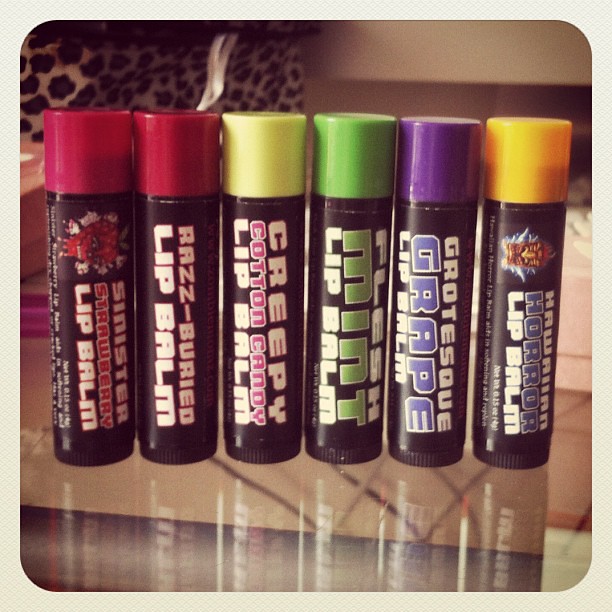This image captures a close-up of six distinct tubes of lip balm arranged neatly on a glass table, their reflections visible on the surface below. Each lip balm tube features a dark brown or purplish-brown base with vibrant, distinctively colored caps, and matching color-coded writing. The tubes are lined up from left to right with the following cap colors: dark pinkish-red, bright red, yellow, green, purple, and orange-gold. Each tube is adorned with its flavor's branding:

1. "Sinister Strawberry Lip Balm" with a dark pinkish-red lid, featuring a brown tube and white and red lettering with an image of a strawberry.
2. "Raspberry Lip Balm" with a red cap, marked with red and white text and a raspberry illustration.
3. "Creepy Cotton Candy Lip Balm" with a yellow top, adorned with white and red font.
4. "Flush Mint Lip Balm" with a green cap and matching green and white lettering.
5. "Grotesque Grape Lip Balm" with a purple lid, displaying purple and white text.
6. "Hawaiian Horror Lip Balm" with an orange-gold top and a mix of white and blue lettering, accompanied by a small gold emblem.

In the background, a leopard print bag and a white lamp with a white lampshade add context and depth to the scene, enhancing the overall aesthetic of the photograph.